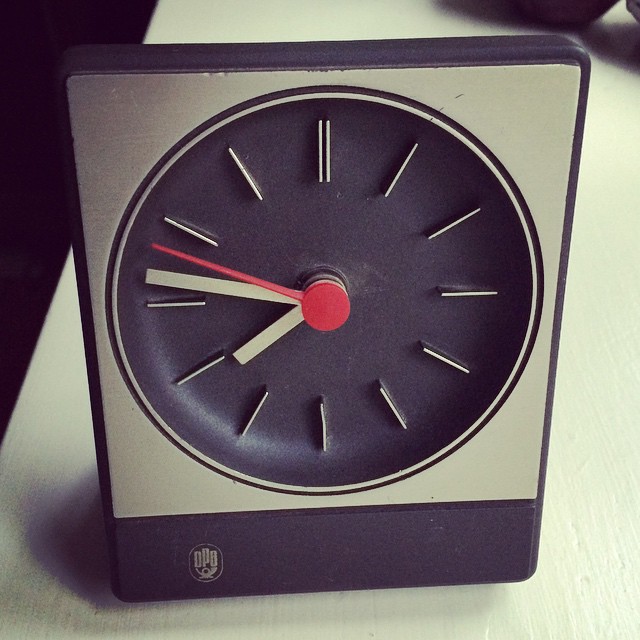This photograph captures a vintage desk clock placed on a white wooden table. The clock, which is primarily beige-colored, stands out with its rectangular shape featuring rounded edges and a stylish design. The clock face is black, showcasing minimalist, white line indicators in place of traditional numbers. The beige minute and hour hands, along with a striking bright red second hand, complement the overall aesthetic. Centrally, the clock has a unique design of a circular stripe pattern, adding to its vintage appeal.

The clock's frame is square-shaped with a metallic, silver background, bordered by a sleek black edge. At the bottom of the frame, a black rectangular section bears the logo "DPO," accompanied by a small symbol that could be interpreted as a horn or two swords. This detail is positioned on the bottom left.

In the upper right-hand corner of the image, there is a dark object casting a shadow, which adds a mysterious element to the scene. Meanwhile, the edge of the floor visible on the left side of the picture appears to be a dark, almost black shade. The combination of these elements makes for a striking contrast against the clean, white wooden table, enhancing the visual appeal of the vintage desk clock.